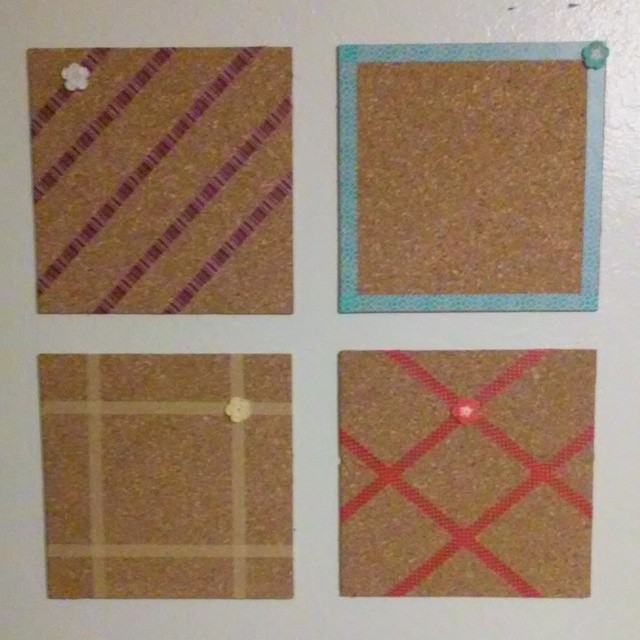This color photograph depicts four square pieces of brown cork board arranged in a 2x2 grid on a light gray or white wall. Each square exhibits a unique decorative pattern with washi tape and has a small flower accent. 

The upper left cork board features five diagonal purple stripes of washi tape extending from the top left corner towards the bottom right, interspersed with the brown color of the cork board. A small white flower is situated in the upper left corner, overlapping some of the stripes. 

The upper right cork board is bordered with blue washi tape and has a matching blue flower with a white center in the upper right corner. 

In the lower left, the cork board is decorated with horizontal and vertical yellow washi tape strips arranged in a window frame or tic-tac-toe pattern. A yellow flower with a white center is attached to the right vertical strip.

Finally, the lower right cork board showcases a criss-cross pattern made of red washi tape. One diagonal red tape runs from the middle of the left side to the top right corner, and another runs from the bottom middle to the right side middle. A red flower is positioned at the intersection of the first two red lines in the top center area.